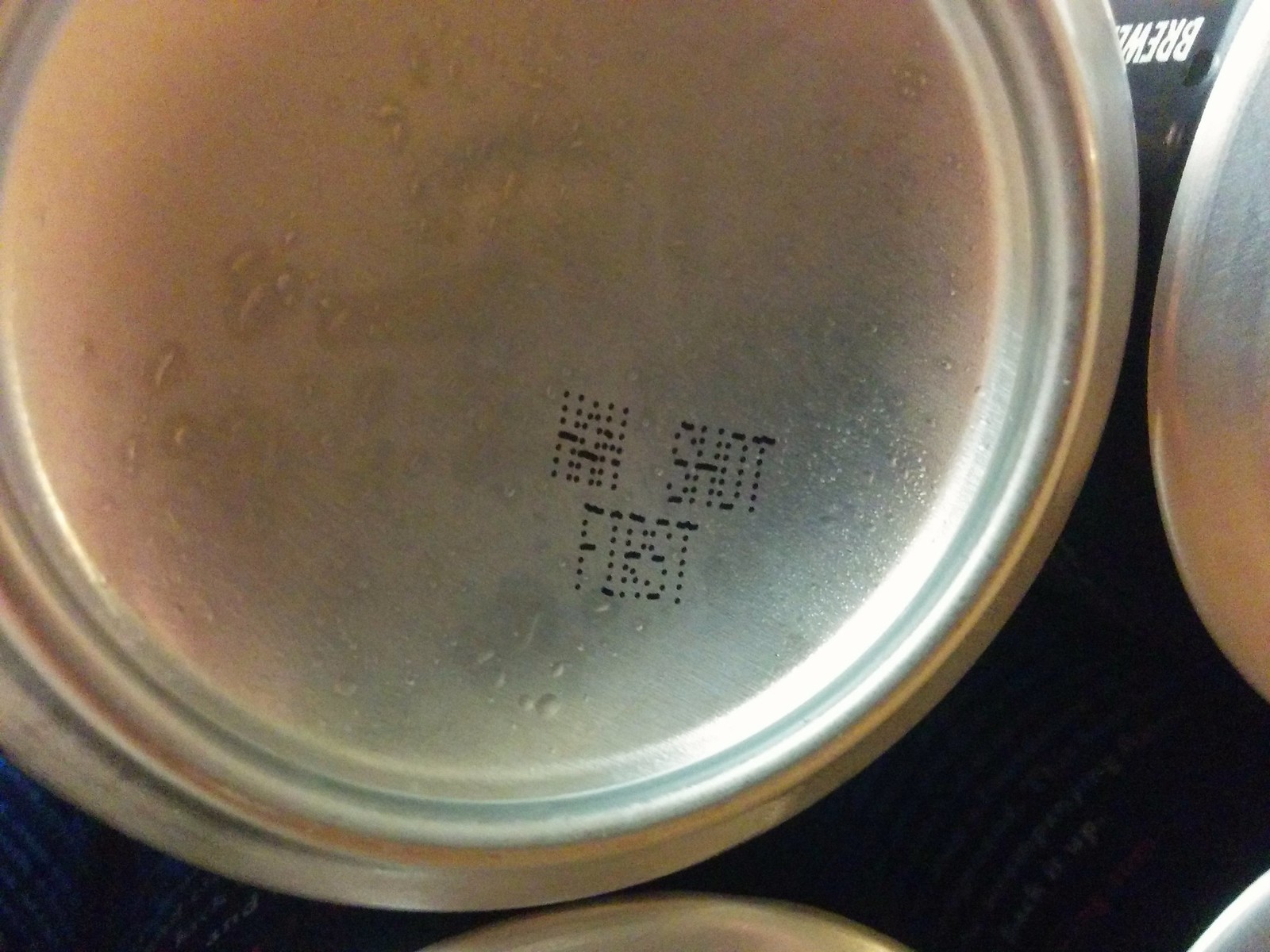This image captures the underside of four aluminum cans, primarily focusing on the bottom of one can. The cans, likely containing beer judging by the partial word "brew," exhibit a frosted, moist appearance, with visible condensation and water droplets. The main can in the foreground prominently displays the phrase "Han shot first" in black dot lettering on its domed, reflective base. The surrounding cans, which are silver with some black and white accents, contribute to a cool, slightly reflective aesthetic, hinting at their cold temperature. This angled shot appears as if taken from beneath a glass surface or shelf, giving a unique perspective on the chilled beverages.